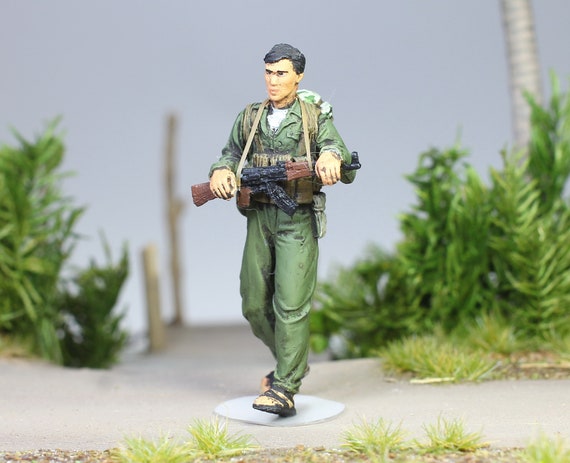This detailed photograph captures a highly realistic diorama featuring a meticulously painted plastic soldier figurine standing at the intersection of a T-shaped concrete path. The soldier, positioned centrally, is depicted in mid-step, wearing black sandals, green military pants, and a green jacket. Over his jacket, he carries beige material, likely supplies, and the top of a white and green backpack is visible over his shoulder. The soldier has pale skin, black eyebrows, black hair, and is holding a black and brown assault rifle, identified as an AK, across his body with a strap over his neck. His hands rest on the gun as if bracing it like a baton.

The background of the image is intentionally blurred to enhance the focus on the soldier, creating depth in the scene. To the left and right edges of the path, the diorama is adorned with miniature leafy plants and the segmented trunk of an unfinished palm tree on the right side. Small tufts of grass are spread along the path's border at the very bottom of the image. The overall scene gives the impression of a verdant, albeit miniature, environment, adding to the realism and complexity of the diorama.